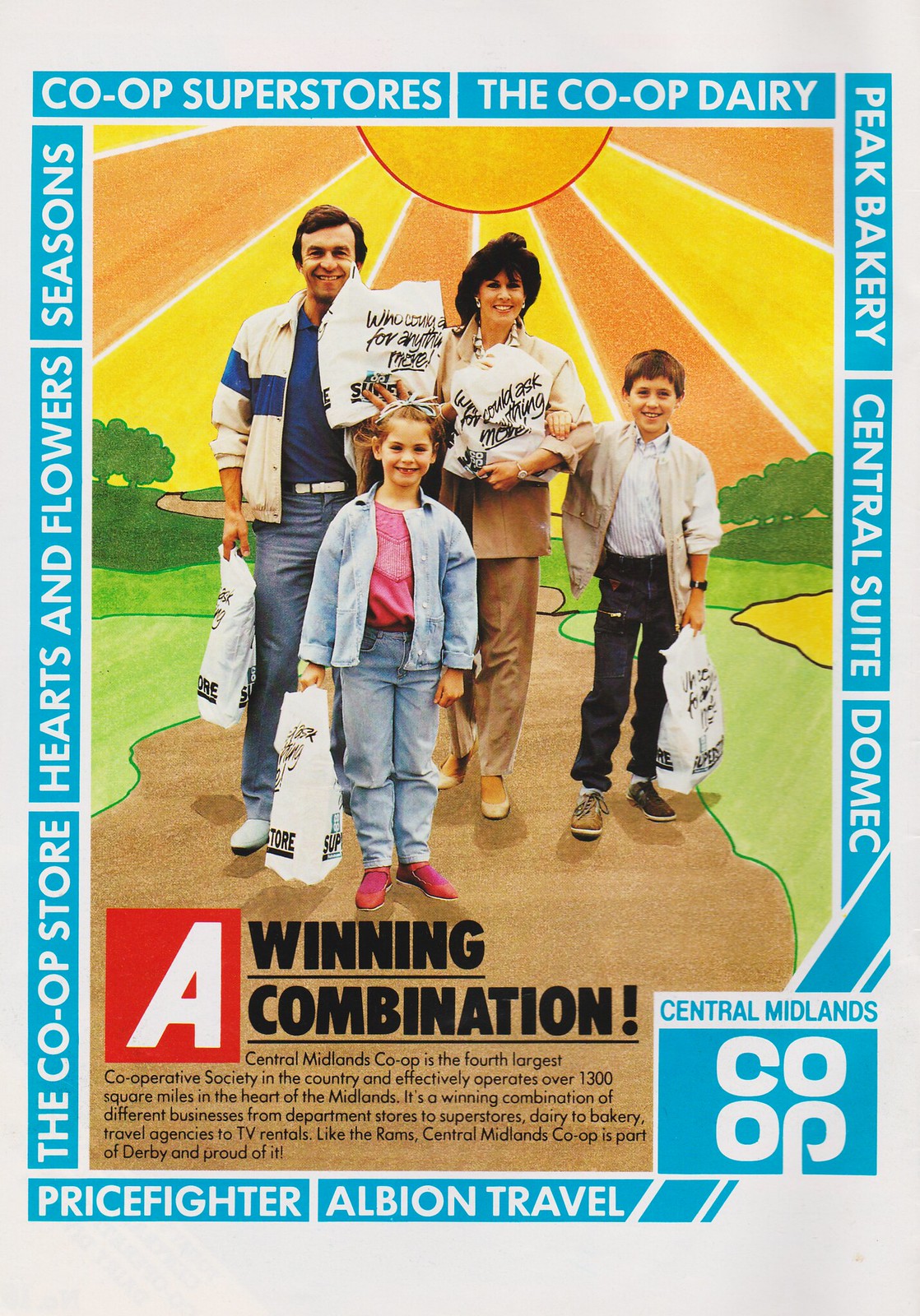This vintage advertisement poster for a food co-op features a real-life family—a mother, father, young boy, and young girl—on a hand-drawn cartoon walking path and background. The family is depicted holding bags of groceries, surrounded by a blue border with text naming different businesses: Co-op Superstores, The Co-op Dairy, Peak Bakery, Central Suite, Domecq, Price Fighter, All Beyond Travel, The Co-op Store, Hearts and Flowers, and Seasons.

At the center of the advertisement, a large red square with white and black bold text declares "A Winning Combination." Below, it reads, "Central Midlands Co-op is the fourth-largest cooperative society in the country and effectively operates over 1,300 square miles in the heart of the Midlands. It's a winning combination of different businesses, from department stores to superstores, dairy to bakery, travel agencies to TV rentals. Like the Ram, Central Midlands Co-op is part of Derby and proud of it." In the bottom right corner, "Central Midlands Co-op" is prominently displayed in blue and white font against a blue background.